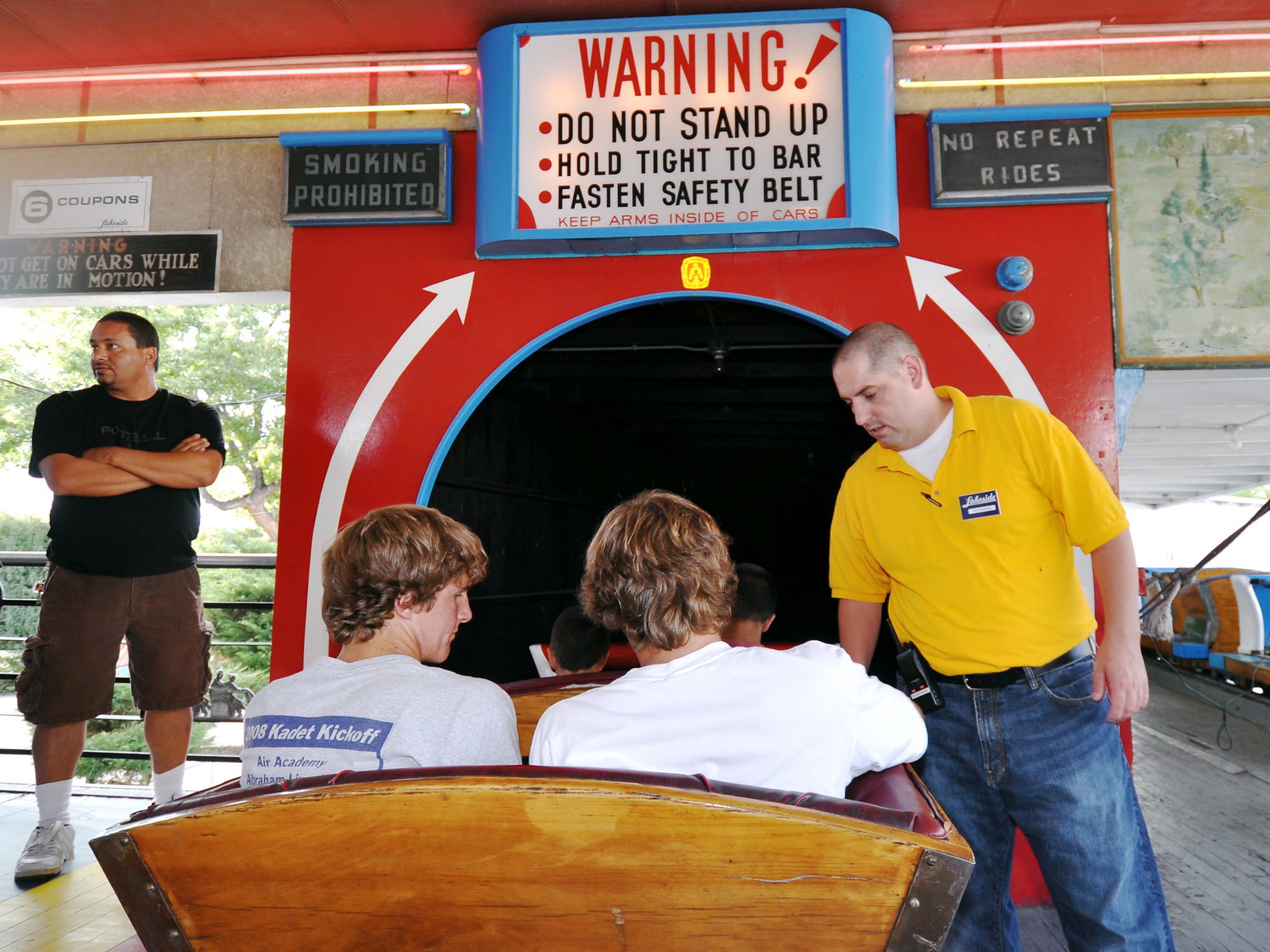This vivid color photograph, taken in landscape orientation during daytime, captures the entrance of a thrilling amusement park ride. In the foreground, we view the backs of two young men with sandy brown hair, wearing t-shirts, as they sit in a golden-hued wooden boat, preparing to enter a black tunnel outlined in a bluish color. The exterior of the tunnel entrance is marked by a shiny red border. Both riders appear relaxed, with one wearing a plain white shirt and the other in a white shirt with blue print.

On the left of the image stands a man with brown skin, his arms folded, dressed in a short-sleeved black shirt, brown shorts, and white sneakers, seemingly waiting and looking to the left side of the frame. To the right, a Caucasian male attendant, identified by his yellow short-sleeved polo shirt over a white t-shirt and blue jeans, is seen bending over the railing, adjusting parts of the ride with a radio attached to his waist.

The tunnel entrance features several prominent signs. An overhead white sign with red letters warns, "WARNING!" followed by black text listing three safety instructions: "Do Not Stand Up," "Hold Tight to Bar," and "Fasten Safety Belt," with an additional caution in smaller red letters to "KEEP ARMS INSIDE OF CARS." On the top left, a gray-lettered sign commands, "SMOKING PROHIBITED," while the right side warns, "NO REPEAT RIDES."

Further away on the right side of the image, there is a row of additional train cars. The surrounding area appears to be an indoor theme park, as indicated by the large undercovering and the warm, diffused daylight filtering through. This scene embodies a rich, detailed slice of amusement park excitement and order.